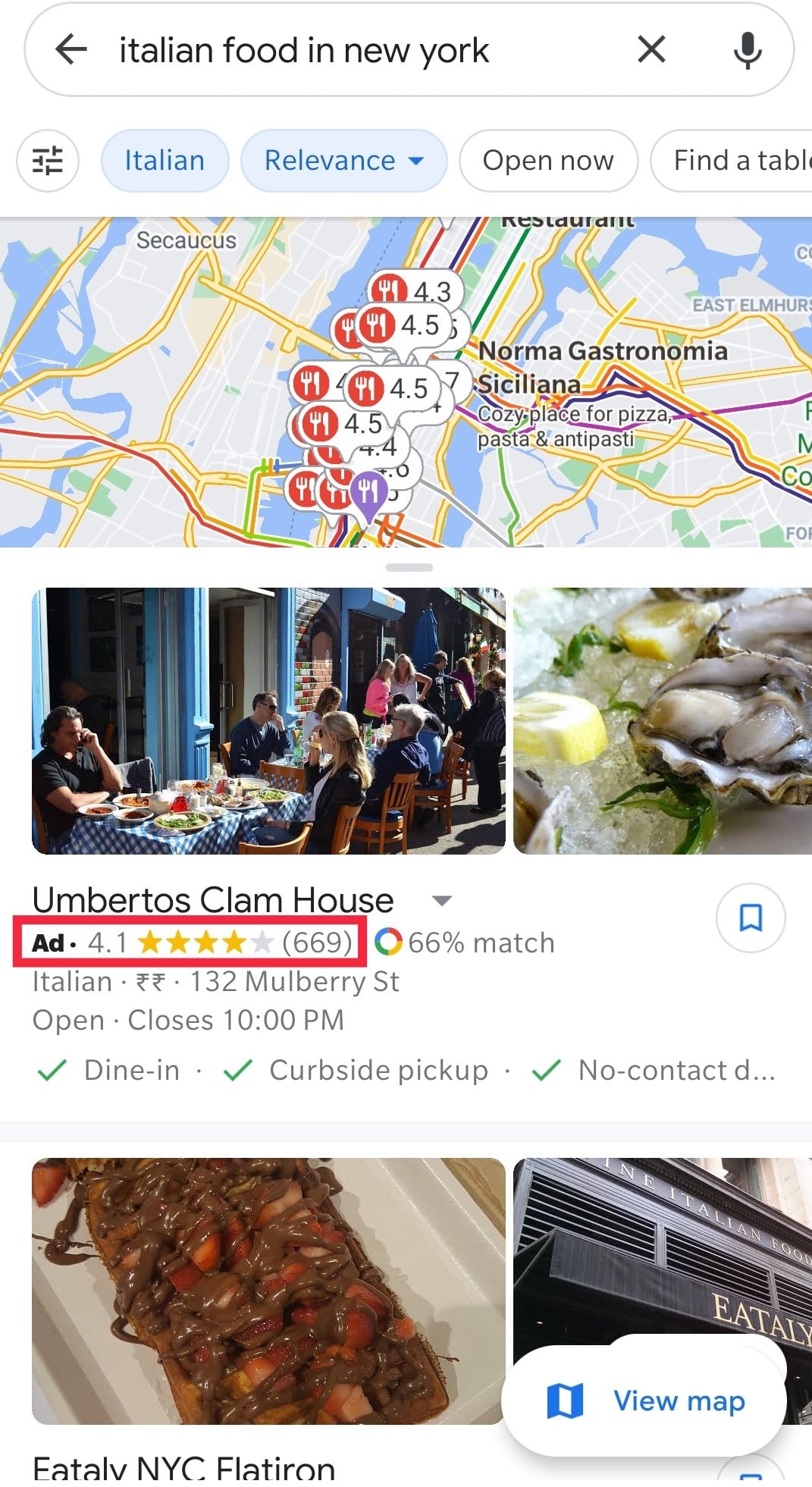A screenshot from a mobile device displays a detailed search on Google Maps for Italian food in New York City. The dark text stands out prominently against a light background, providing clear visibility. The search filters, conveniently presented as bubbles, show 'Italian' and 'Relevance' as selected options, signifying a refined and specific search. Other available but unselected filters such as 'Open now' and 'Find a table' remain highlighted in white with dark text.

Beneath the filters, the map of New York City is peppered with numerous restaurant icons, indicating the dense availability of Italian eateries in the area. Highlighted prominently in the results is 'Umberto's Clam House', which boasts a four-star rating. Accompanying this listing are two distinctive images: on the left, a group of people are seen dining outdoors at a table adorned with a blue checkered tablecloth, capturing a convivial and inviting atmosphere. The adjacent image on the right is a close-up shot of freshly served oysters, showcasing the restaurant's seafood offerings.

Further down, additional information about Umberto's Clam House is presented in a concise manner, detailing their services that include dine-in options, curbside pickup, and no-contact delivery. The bottom section features two more images; the left image portrays a delectable dish, though it is unclear whether it is a dessert or a savory meal. The right image displays the restaurant's inviting facade, offering a glimpse of what patrons can expect before stepping inside.